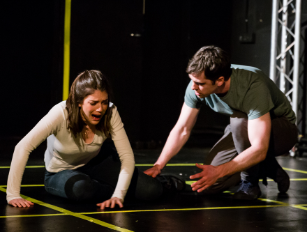The photograph captures a dramatic scene against a black background, possibly on a stage or a game floor delineated with thin yellow lines. On the left side, a woman with dark brown, shoulder-length hair is sitting on the black floor with her hands placed in front of her. She appears to be in pain, her mouth open and eyes cast downward, seemingly crying or shouting. She is dressed in a long-sleeve tan shirt and dark pants. To her right, a man with short black hair, clad in a green t-shirt and gray pants, is crouching close to her, extending his arms in a consoling gesture. He places one hand gently on her leg, his facial expression marked by concern and a desire to help. The image poignantly captures a moment of emotional distress and empathy.